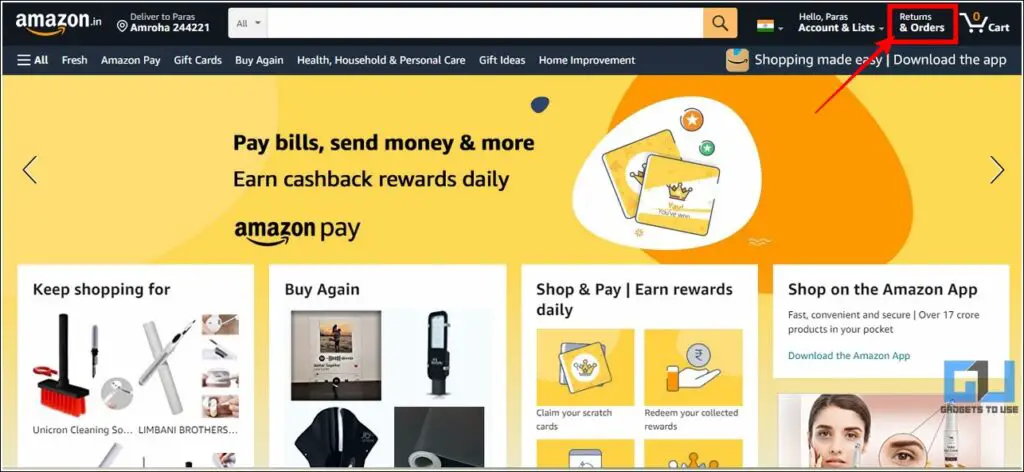This detailed caption describes the elements in a screenshot of the Amazon.in website, emphasizing the various components visible on the page:

---

The image is a detailed screenshot from the Amazon.in website. The topmost section features a dark bluish navigation bar. On the left-hand corner of this bar, the Amazon logo is prominently displayed with the curved arrow extending from 'A' to 'Z'. Right next to the logo, it reads "Delivered to Paris, Amroa, 244-221". Centrally located, there's a search bar. To the left of the search bar, a dropdown menu currently set to "All" is visible, while to the right, the magnifying glass icon represents the search function. Adjacent to the search bar, there's an icon of the Indian flag. Further along the bar, the text "Hello, Paris, Account & Lists" appears, followed by "Returns & Orders". Superimposed on the screenshot, a red box with an arrow highlights the "Returns & Orders" button. On the extreme right, there's the cart icon, which currently shows '0' items.

Below the dark blue bar, another lighter-colored bar runs horizontally across the page. On the left of this bar, a burger menu labeled "All" is displayed. To the right are several sections: "Fresh", "Amazon Pay", "Gift Cards", "Buy Again", "Health, Household, and Personal Care", "Gift Ideas", and "Home Improvement". Further to the right, it mentions "Shopping made easy, download the app". 

Beneath this, a promotional banner says "Pay bills, send money, and more, earn cashback rewards daily with Amazon Pay". At the bottom section of this screenshot, several categories are listed such as "Keep Shopping For", "Buy Again", "Shop and Pay", "Earn Rewards Daily", and "Shop on the Amazon App".

---

This caption clearly describes each element, providing a detailed overview of what is depicted in the screenshot.